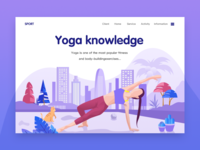This image showcases the home screen of a website. The composition is compact, with the background surrounding the website interface on the top, bottom, left, and right sides. The background transitions from a lighter purple color at the top to a blend of blue and purple below. The main background of the website itself is white.

In the top left corner of the website, the name of the site is displayed, followed by five categories arranged horizontally to the right. Below these categories, the text "yoga knowledge" appears in blue, and underneath that, there's a descriptive sentence in gray text.

The central design features an animated person performing a yoga pose, balancing with one hand on the ground and the other hand raised. This animated figure has long hair styled in a ponytail that almost touches the ground. The character is dressed in purplish-colored pants and a blue top, set against a backdrop with buildings and trees. The visual includes four trees—two with blue foliage and two with pink leaves.

Additionally, a yellow animal is positioned to the left of the yoga figure, while two houseplants in vases are placed to the right. The base of the ground is mainly white, completing the overall simple yet aesthetically pleasing sketch and design of the website.